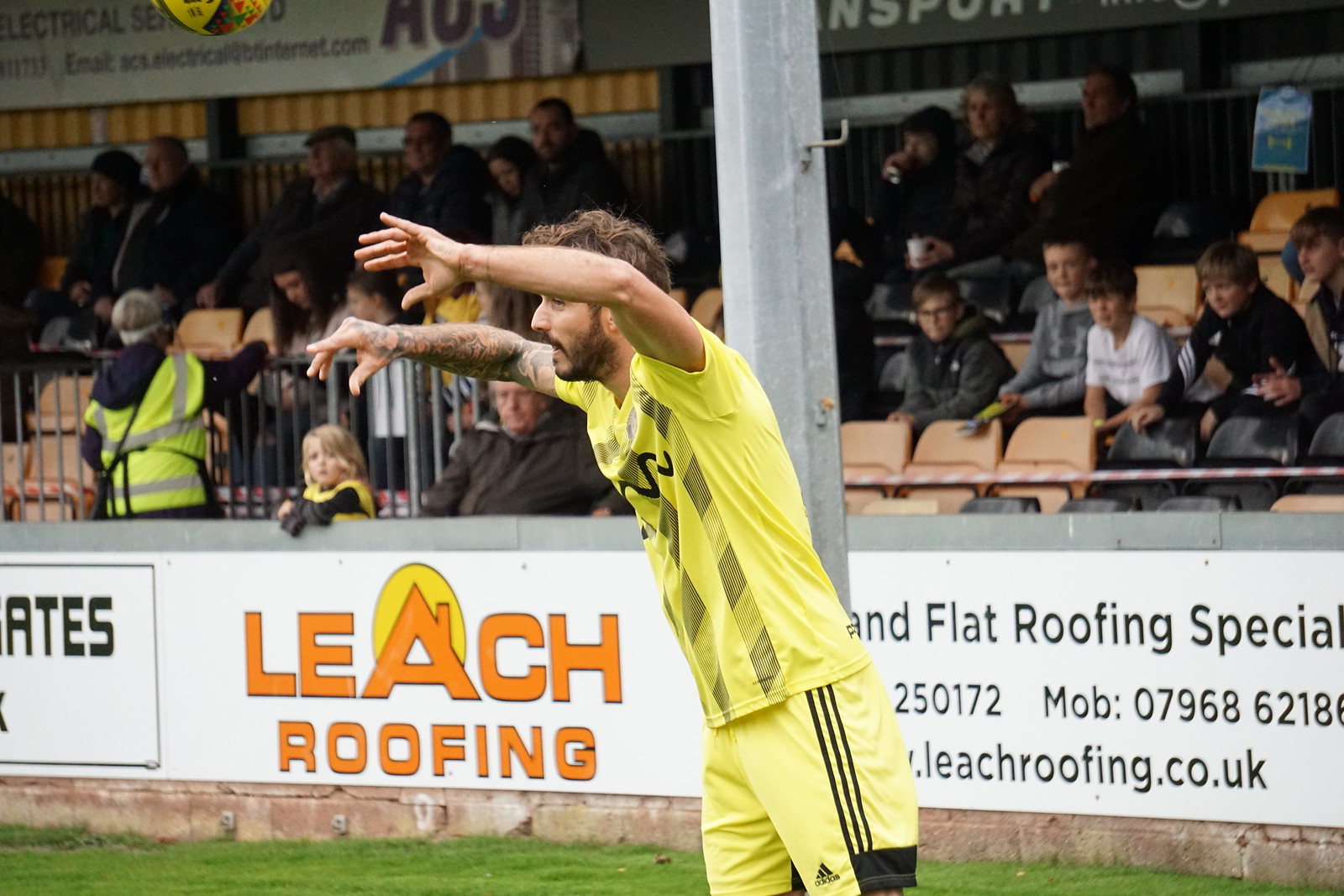In this image from a British football game, a male athlete in a black and neon yellow uniform is prominently featured with his arms raised and leaning slightly forward. The player has light brown hair, a beard, and a mustache, along with tattoos covering his right arm. The scene is set on the field, and behind the athlete is a spectator stand with a mix of adults and children, some seats filled and others empty. A wall dividing the field from the spectators carries advertisements, notably one for Leech Roofing, featuring text that reads "flat roofing special 250172, mob 0796862186, leechroofing.co.uk," although partially obscured by the player and a pole. The colors present in the image include yellow, peach, green, brown, orange, white, and black, adding vibrancy to the casually taken photo, likely shot by a professional on the field.